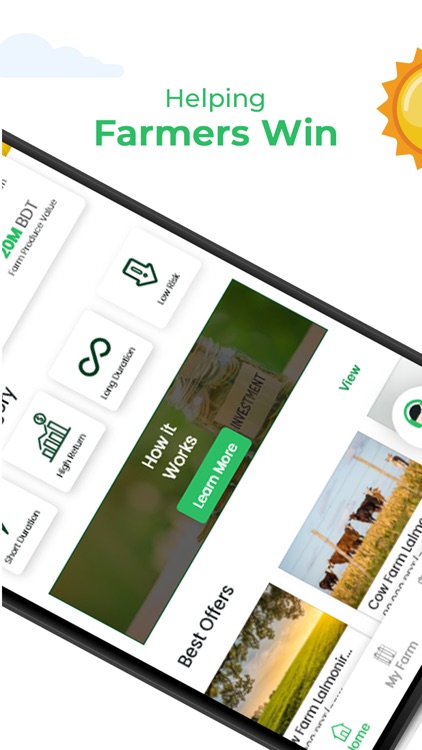This graphical poster, styled as an advertisement for a mobile phone application, features a clean white background. A grey cloud decorates the top left corner, while a vibrant graphic sun shines from the top right. Prominent green text in the center of the poster proclaims, "Helping Farmers Win." 

Taking center stage, a smartphone is depicted lying horizontally across the screen at a slight angle. The device's screen, partially cropped at both the top and bottom, displays the interface of the application being advertised. 

Icons within the application suggest various investment options, including "Short Duration," "High Return," "Long Duration," and "Low Risk." Another section titled "How it Works" features a green button labeled "Learn More." 

Overall, this poster appears to promote an application designed for investing in farming stocks, emphasizing ease of use and lucrative opportunities for farmers and investors alike.